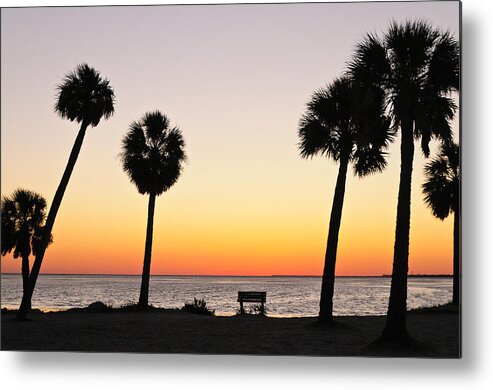The image is a stunning canvas print of a tranquil beach scene captured at sunset. In the foreground, a solitary bench sits serenely on the sand, centrally positioned and facing the vast expanse of the ocean. This bench is flanked by six towering palm trees, three on each side, their fronds silhouetted starkly against the evening sky. As the horizon meets the water, the sky is awash with a gradient of colors: deep orange at the horizon, transitioning softly into yellow, which then fades gently into a pale white-blue as it reaches the upper edge of the image. A distant landmass is barely visible on the right-hand side of the horizon, adding a subtle detail to the scene's composition. The beach itself is almost devoid of movement; even the ocean is still, mirroring the sky's fading hues. The overall mood is one of stillness, peace, and quiet reflection, devoid of people or any signs of wind. This landscape-format photograph perfectly captures a moment of serene beauty, making it a compelling piece of art.